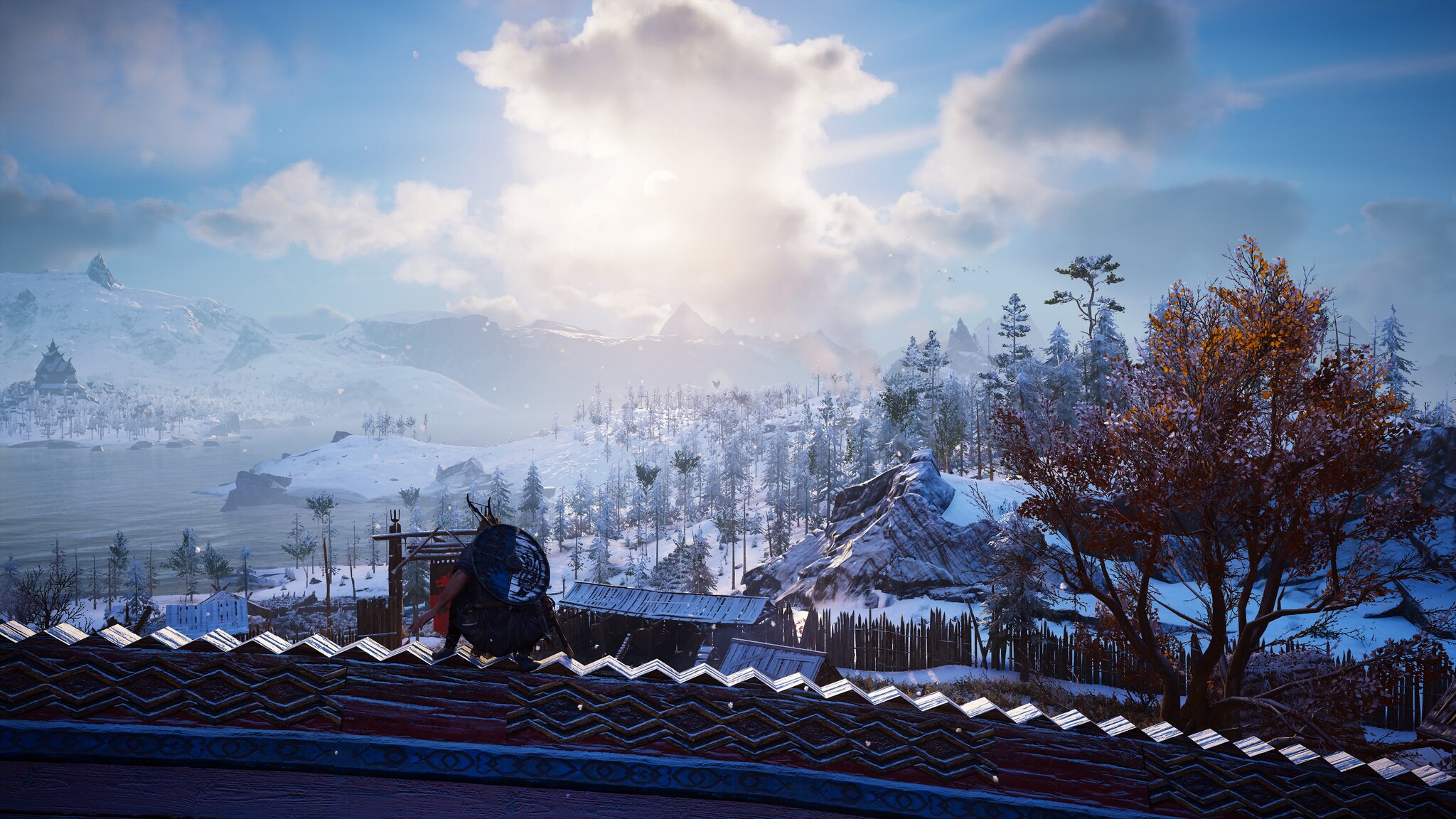Amidst a serene winter landscape, the image depicts a scene reminiscent of either a painting or intricate video game graphics. Snow-covered mountains dominate the background, with numerous evergreen trees blanketed in white. The sky is a blend of bright clouds partially obscuring the sun, casting a bluish tint over the terrain. 

In the foreground, a figure is crouched on a rooftop, facing away from the viewer. Clad in medieval attire, he bears a round wooden shield adorned with blue and white patterns, suggesting a Viking or possibly samurai warrior. A helmet tops his head and a bow and quiver are strapped to his back, indicating his readiness for a potential hunt or ambush.

The setting is rich with detail: a reddish-brown tree adds a splash of color amidst the monochromatic snow, and rustic brown fencing outlines the area. Below, an icy river winds through a snow-laden village of wooden houses, their roofs heavily covered in snow. The entire scene evokes a sense of historical tranquility, underscored by the warrior's vigilant stance against the backdrop of an old-fashioned winter village.